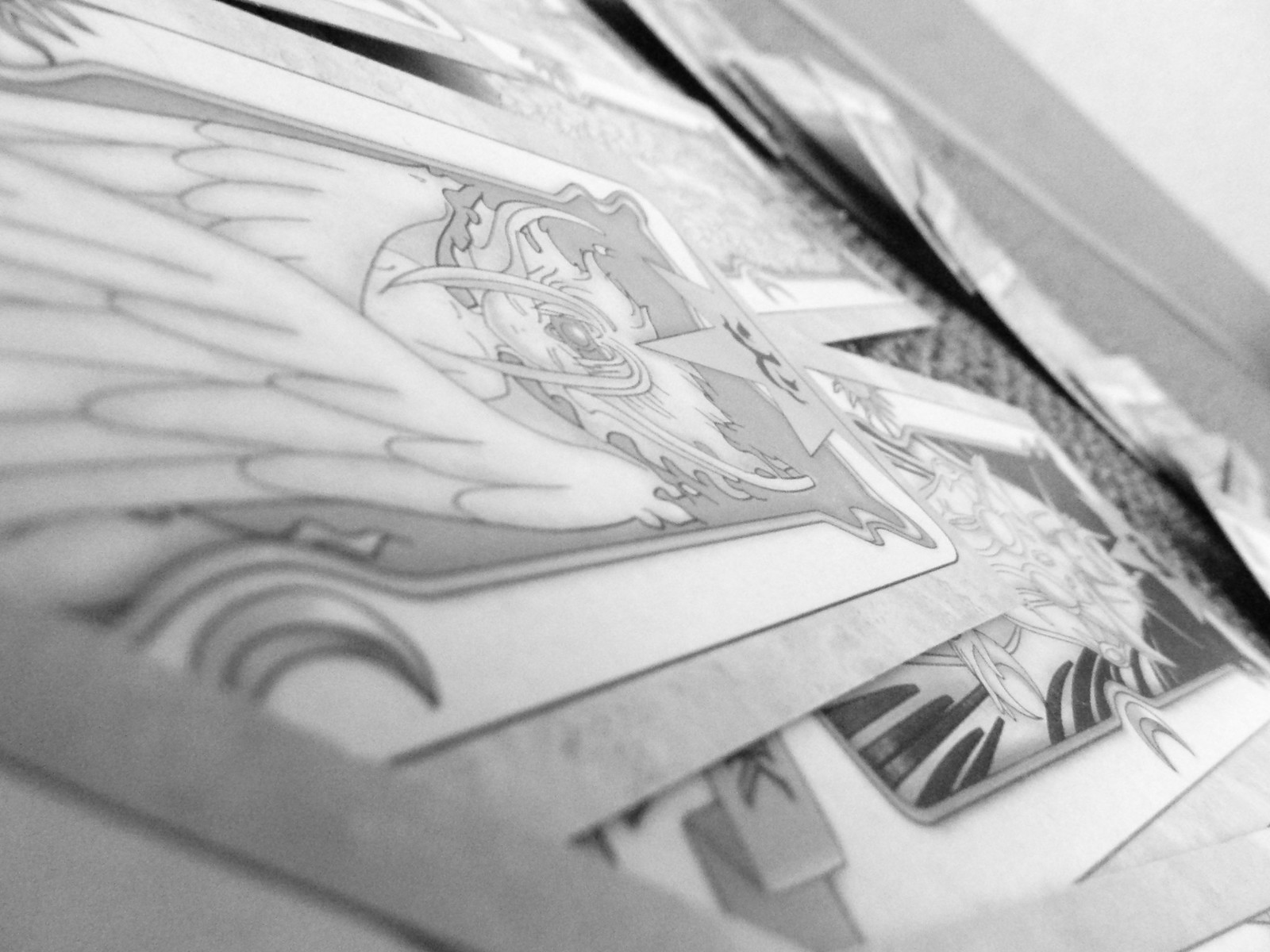A detailed black and white photograph captures a close-up view of what appears to be a collection of Pokémon or anime-style cards scattered on a textured Berber carpet. The cards are haphazardly spread out, with one prominently displaying an illustration of a moon. Another card features a girl adorned with wings that appear to be folded around her, with a round emblem situated between her closed eyes. Beneath this card, another character is partially visible, resembling a rat. This card also includes a moon motif, adding a mystical element to the monochromatic scene. The lack of color accentuates the intricate details of the illustrations and the textures of the carpet.